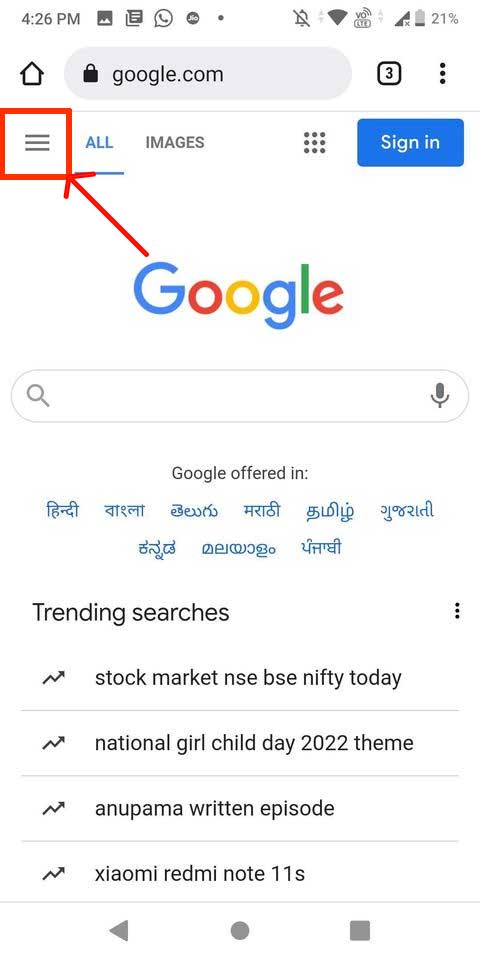A smartphone screenshot taken at 4:26 PM displays a detailed view of the device's home screen and a Google search page. At the top of the screen, status icons for sound (off), Wi-Fi, VoLTE, and a battery level at 21% are visible. Below these, there are multiple app icons, including pictures, documents, WhatsApp, and an indiscernible one, with the camera icon centered. 

The bottom navigation bar features a home icon and a Google.com search box showing "google.com." Three tabs appear with a three-dot vertical menu. 

A red arrow highlights important elements, starting at the Google logo, pointing to a hamburger menu in a red box, and moving right to tabs labeled "All," "Images," "Apps," and a blue "Sign In" button.

Further down, the central Google icon is followed by a search box and a microphone symbol. Beneath this, Google offers various language options that are not clearly specified. Trending searches are listed vertically, each preceded by a squiggly arrow. The entries include: 
- "Stock market, NSE, BSE, Nifty today"
- "National Girl Child Day 2022 theme"
- "Anna Palma written episode"
- "Xiaomi Redmi Note 11S."

Finally, the screen's bottom features navigation buttons for back, home, and recent apps.